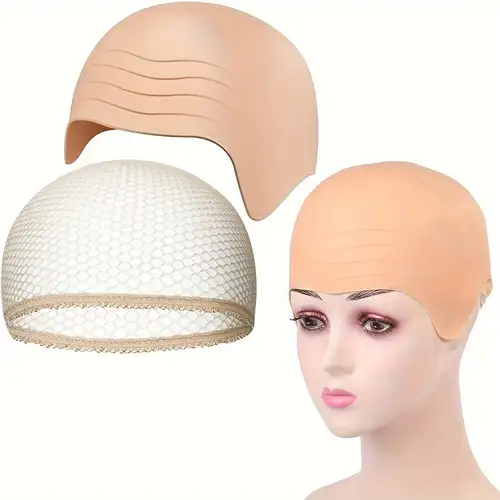This detailed illustration features a female-faced mannequin head on the right side of the image. The mannequin is adorned with vivid makeup, including light pink lipstick, pink eyeshadow around the eyes, black mascara, and dark, drawn-on eyebrows. Her slim face appears to lack ears, and her eyes are wide and staring. The mannequin's closed mouth and long, smooth white neck give her a distinctive look. Covering her head is a neutral rubber cap, characterized by four prominent lines on the forehead, contributing to a bold and structured appearance. Below this cap, there is a net-like part that is white and green with brown tones underneath. Her head is slightly tilted downward, adding a subtle grace to the otherwise stark and expressive presentation.